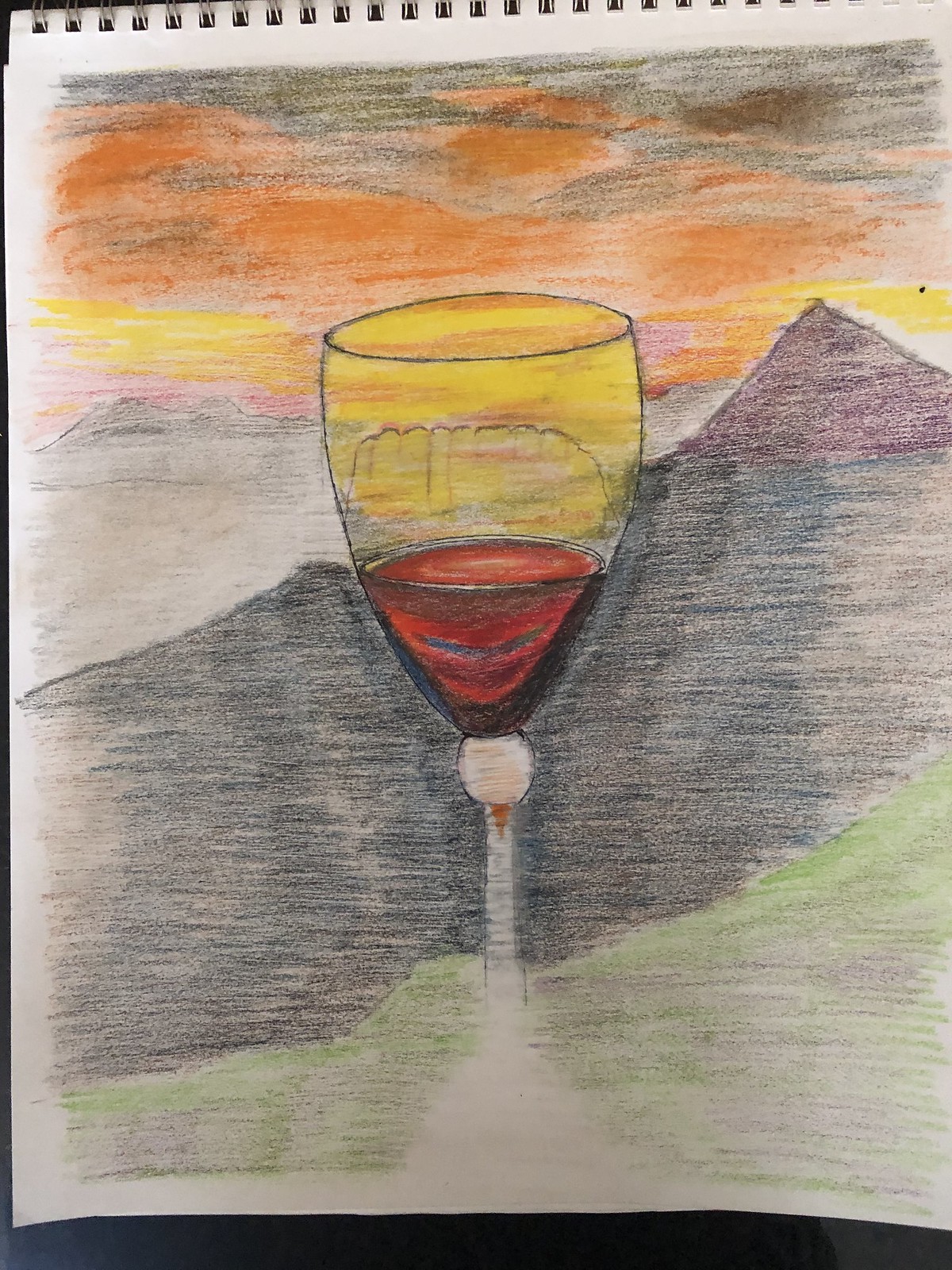In this vibrant and intricate drawing displayed on a sketch pad, the focal point is a meticulously rendered glass of red wine with an elegant, elongated stem. The lower third of the glass is filled with a rich, deep red liquid, capturing the subtle reflections and hues characteristic of fine wine. The backdrop of the artwork is a vivid and layered landscape: the base features lush, green grass that transitions into rolling, black hills and distant mountains. Beyond these elements lies a gray expanse, suggesting the desolate ground past the mountains, with further mountainous silhouettes receding into the horizon. The sky above is painted in a stunning gradient of orange, yellow, and red, evoking the ethereal beauty of twilight. Contrasting this warm palette, dark, ominous clouds hover near the top of the composition, adding depth and drama to the scene. The overall effect is a striking balance of color and form, creating a mesmerizing visual narrative.